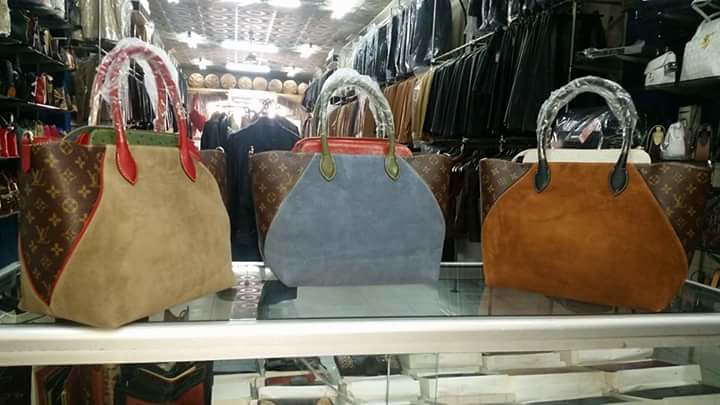This photo captures the interior of a store featuring fluorescent lights on the ceiling and a variety of clothing and accessories on display. On the right-hand side of the aisle, there are racks holding an assortment of coats in shades of black, brown, and tan, commonly worn with suits. The left side of the aisle has another shelf, although the specific items are too small to discern clearly. Dominating the foreground is a clear glass display case topped with three distinctive women's pocketbooks. The first purse is tan and brown with a red strap, the second is light blue and brown with a gold strap, and the third is light brown and dark brown with a black strap. These purses, possibly knock-off Louis Vuitton, feature the brand's logos on the left and right sides with a plain leather patch in the middle. Each handle is in a matching color and wrapped in protective plastic. Reflections on the glass and additional items in the background contribute to the vibrant, bustling atmosphere of the shopping area.